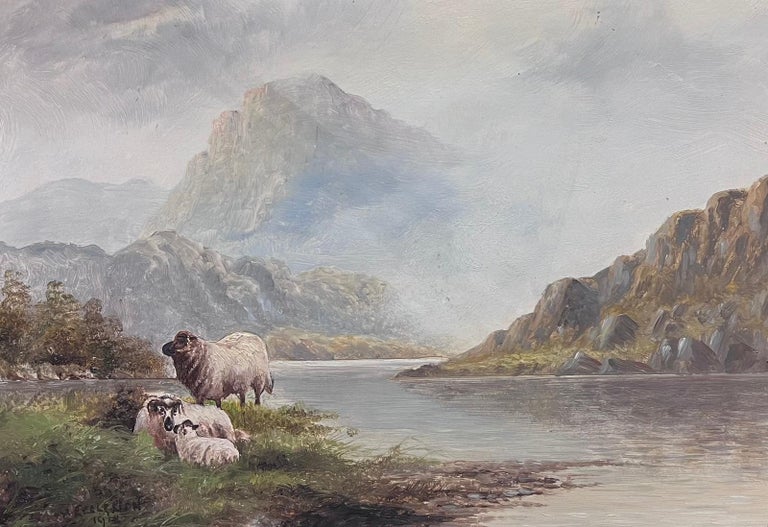This painting captures a tranquil scene featuring a family of mountain sheep by a slow-moving, winding river in a very mountainous and rocky landscape. Dominated by muted greens, grays, blues, and browns, the image portrays a tall, imposing mountain in the background with smaller hills on the sides, all cloaked in misty, fog-laden skies. 

In the foreground, on a grassy patch by the river, stands a mother sheep gazing into the distance. Nearby, the father sheep lies comfortably in the grass, while their baby sheep stands facing him, creating a touching family tableau. The mountains and hills are dotted with various rocks and sparse vegetation, contributing to the natural and serene atmosphere of the painting.